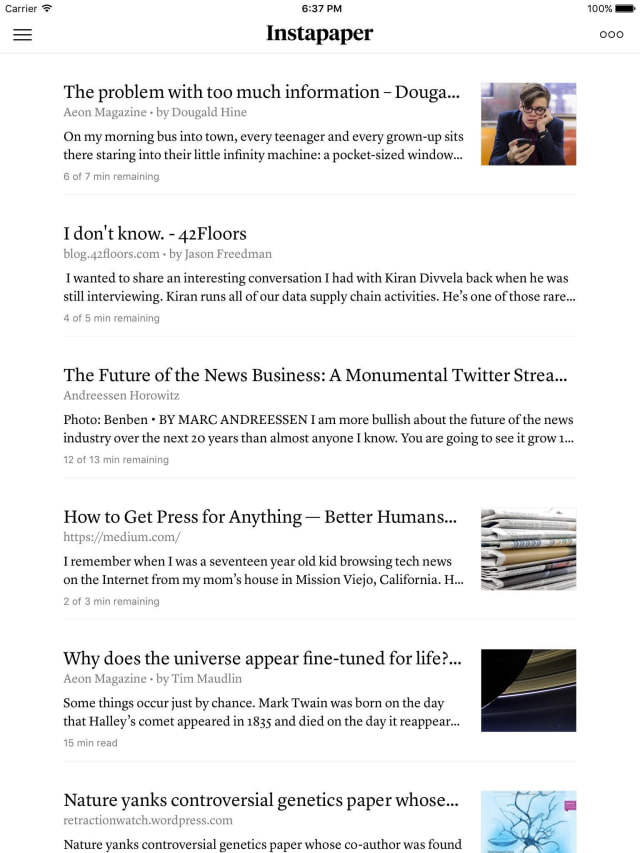This image is a screenshot taken from a cell phone using the Instapaper app, identifiable by the standard phone icons visible in the upper corners of the screen. In the top center, the time is displayed, with the word "Instapaper" prominently featured below it in bold, capitalized black font. The main body of the image displays a list of six articles, reminiscent of search results, each comprising a title, the source, the author, and a brief excerpt.

The first article is titled "The Problem With Too Much Information," sourced from Aeon Magazine, and authored by Dougal Hine. The second listing, titled "I Don't Know," is from the blog "42 Floors" and written by Jason Friedman. The third title on the list reads "The Future Of The New Business," followed by an incomplete mention of "a monumental Twitter," and an unclear source attributed to the letters "S-D-R-E-M" or "S-D-R-E-A" ending with an ellipsis.